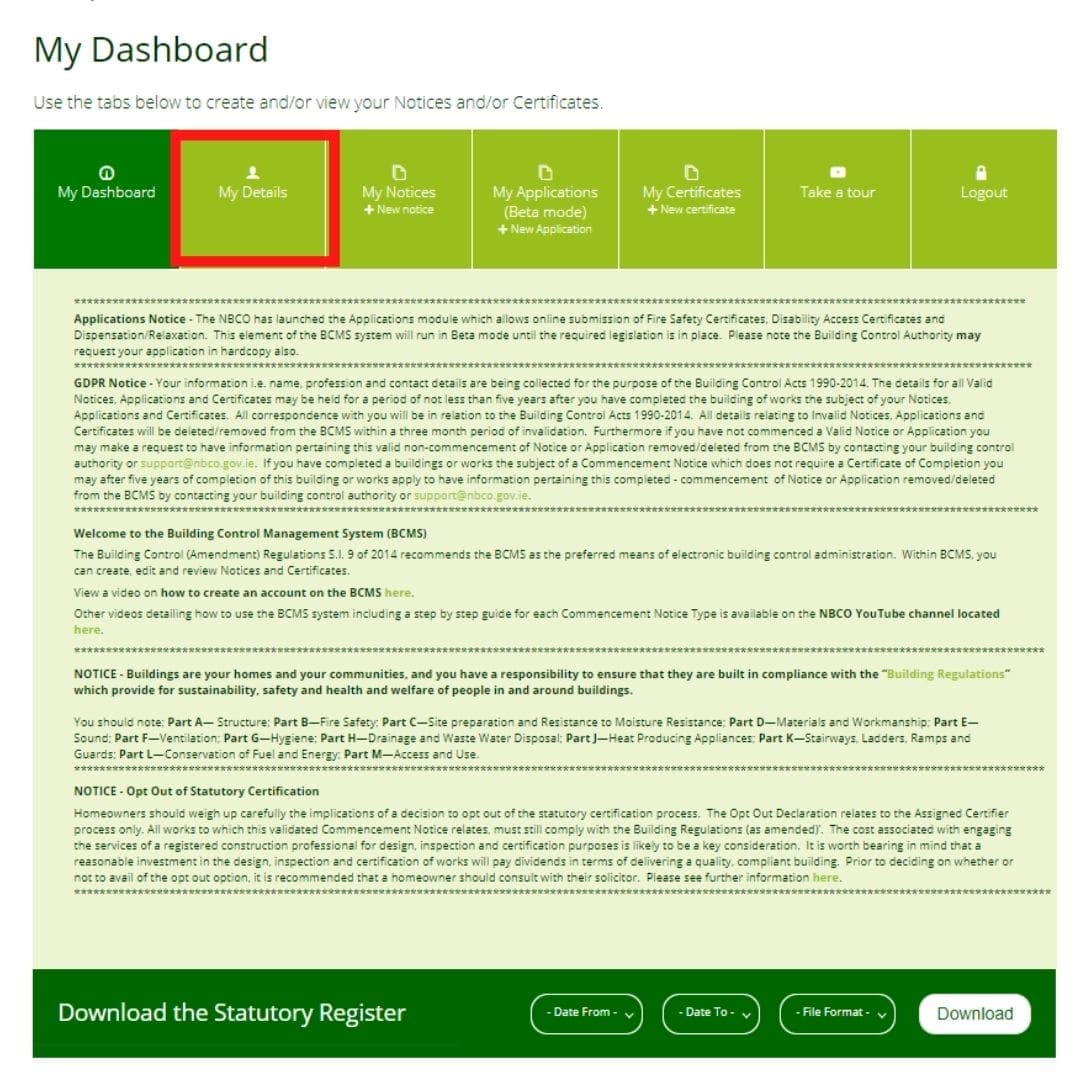This image is a highly detailed screenshot of a user’s dashboard, likely from a building control or compliance management system. At the very top, there is a white horizontal bar with "My Dashboard" displayed prominently in black text. Directly below this, instructional text reads: "Use the tabs below to create and/or view your notices and/or certificates."

Beneath the instructions, there are several buttons in varying shades of green. The darkest green button on the left is titled "My Dashboard," while the adjacent lime green buttons are labeled "My Details," "My Notices," "New Notice," "My Applications (Beta Mode)," "New Application," "My Certificates," "New Certificate," "Take a Tour," and "Log Out."

Following the navigation buttons, the main content area features a pale greenish-gray box titled "Application Notice." The text inside this box explains that the NBCO has launched an application module allowing for the online submission of fire safety certificates, disability access certificates, and dispensation/relaxation requests. It notes that this module will operate in beta mode until the required legislation is established. Users are cautioned that the Building Control Authority might also request a hard copy of their application. Additionally, there is a GDPR notice stating that personal information (name, profession, and contact details) is collected for purposes defined in the Building Control Acts of 1990 to 2014 and may be retained for a minimum of five years following the completion of the relevant building works.

At the bottom of the section, a green bar labeled "Download the Statutory Register" spans the width of the box, accompanied by a white "Download" button on the far right side.